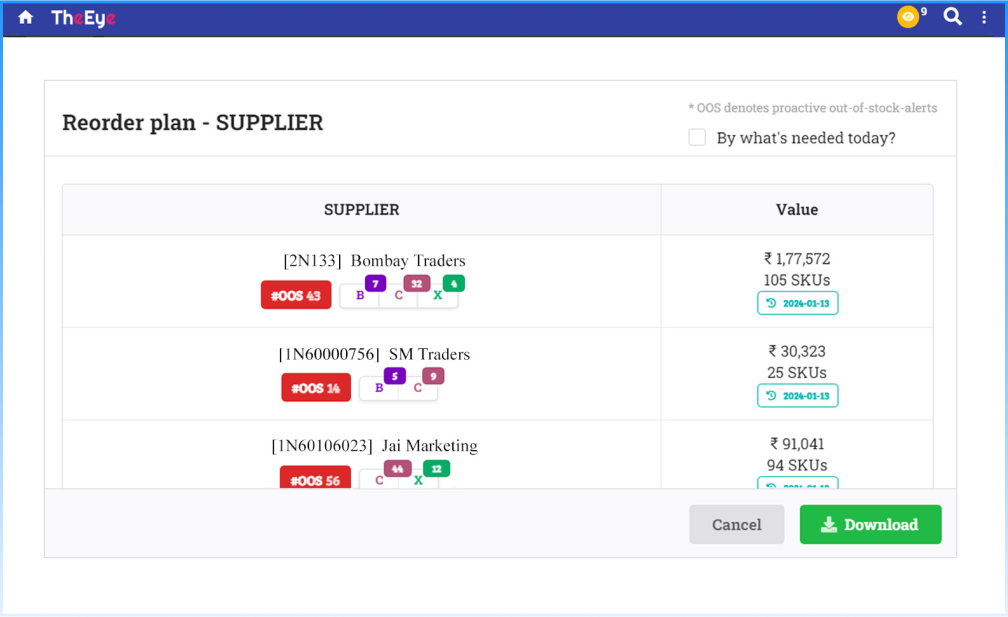The web page features a bright blue ribbon running across the top of the screen. On the left side of the ribbon, there is a white home icon. Adjacent to this, the text "THE EYE" is prominently displayed with the letters 'T,' 'H,' and 'E' in white, while the trailing 'E' in "THE" and the 'E' in "EYE" are in red. 

On the far right side of the ribbon, there is an orange circle containing a white eye symbol, topped by a small number nine, likely indicating a notification. Next to this icon is a magnifying glass, signifying a search function, followed by three vertical dots, presumably for additional options. 

Below the blue ribbon, a white background section hosts a box outlined in a faint gray line. At the top of this box, the text "Reorder Plan - SUPPLIER" is written in black, with "SUPPLIER" fully capitalized. To the far right of this text, there's a small checkbox with gray text next to it that reads, "Buy what's needed today?" 

Beneath this header, the section is divided into two columns: one labeled "Supplier" on the left and the other labeled "Value" on the right.